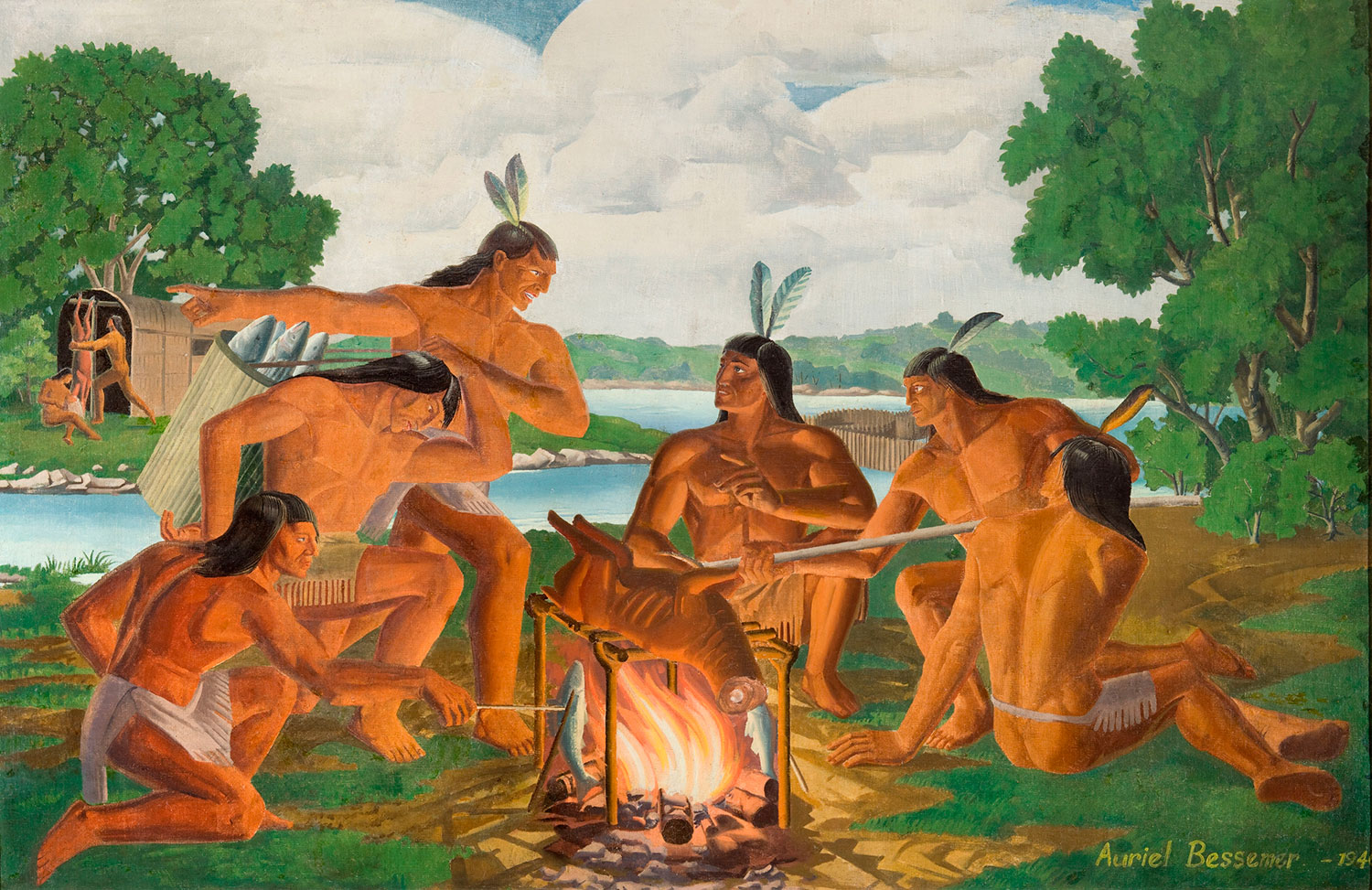This is a detailed color painting by Aurel Bessemer from 1940, depicting a group of six Native American men gathered around a campfire near a river. They are adorned with long black hair, some with feathers, and are dressed in white or brown loincloths. The men are in various positions: seated, standing, and crouching. At the center, a campfire is roasting the torso of a headless four-legged animal, possibly a deer, on a wooden frame. One of the men is holding a fish on a stick over the fire, while another, who has a basket of fish heads on his back, is in conversation with a man in the center. The scene is set against a grassy background with trees flanking the right side and a stream in the background. To the left, a shelter is visible where a man is butchering an animal with a woman sitting nearby, and beyond them, two more men are stringing up another animal by a barrel-shaped structure.